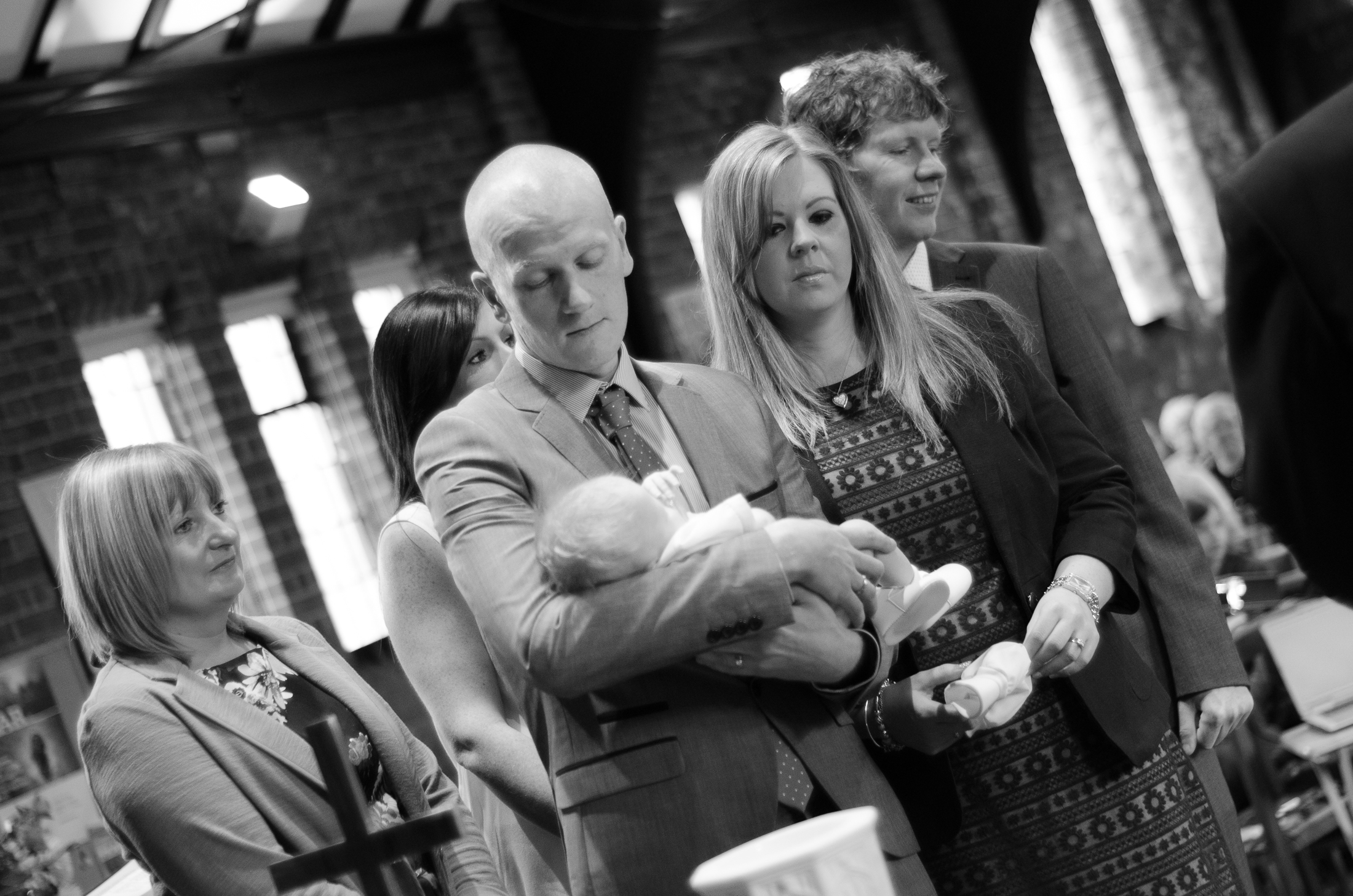In this black-and-white photograph, a formally dressed couple is prominently featured, holding a baby in their arms. The man, who is bald and wearing a suit, gazes down lovingly at the child, while the woman, dressed in a patterned dress with a jacket, stands beside him. Her long, light-colored blonde hair is parted on the side. The couple seems to be at a baptism or a similar church ceremony. 

Several other people are standing behind the couple: a man to the right of the woman and two women to the left of the man. The woman closest to the couple has dark hair and eyes, while the other woman, with lighter-colored hair, wears a light-colored jacket over a dark dress. 

The background is blurred, emphasizing the family, but you can see at least three windows allowing light to stream in, suggesting they are in a brick building with multiple sources of illumination. The setting appears to include church seating with attendees faintly visible. Notably, in the foreground, a cross and a chalice or cup are discernible, adding to the solemn and ceremonial atmosphere. The photograph is taken at a slight angle, making the image appear slightly tilted.